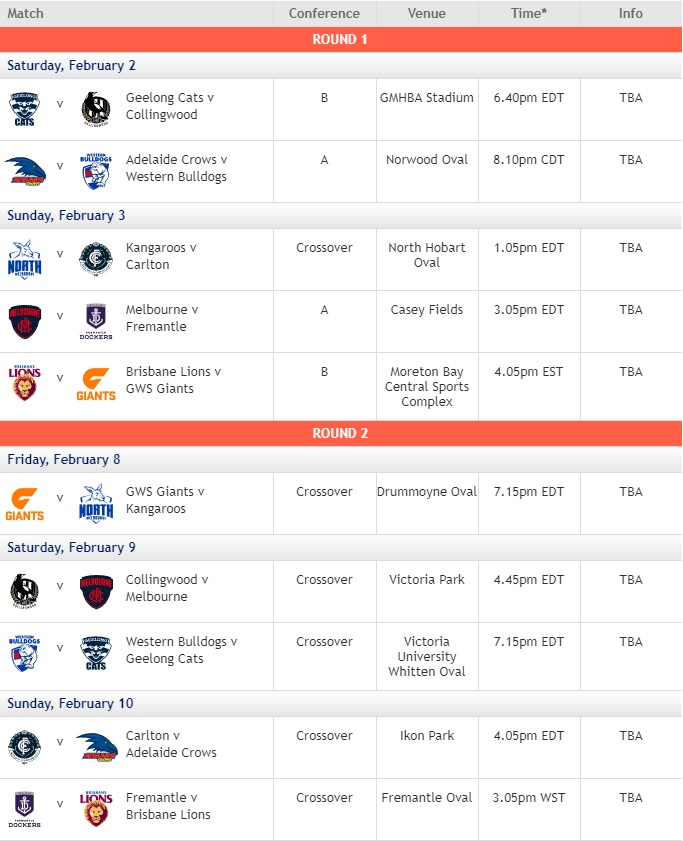This screenshot features a detailed schedule for various sports teams, likely basketball, as indicated by the context. The teams listed include the Giants, Lions, Bulldogs, among others. At the top of the page, several column titles organize the information. 

1. **Match** - The first column, titled "Match," lists the teams competing against each other and the dates of their matches. 
2. **Conference** - This column indicates the group each team belongs to, such as Group A or B.
3. **Venue** - The location where each game will be held.
4. **Time** - The scheduled start time for each game, noted with an asterisk suggesting the times might be subject to change.
5. **Info** - This column predominantly contains "TBA," signaling that additional information is yet to be announced.

The schedule begins with games on Saturday, February 2nd, featuring matches between Geelong Cats vs. Collingwood and Adelaide Crows vs. Western Bulldogs. Other matches are scheduled for February 3rd, 8th, 9th, and 10th, but specific details for these dates are also included in the table.